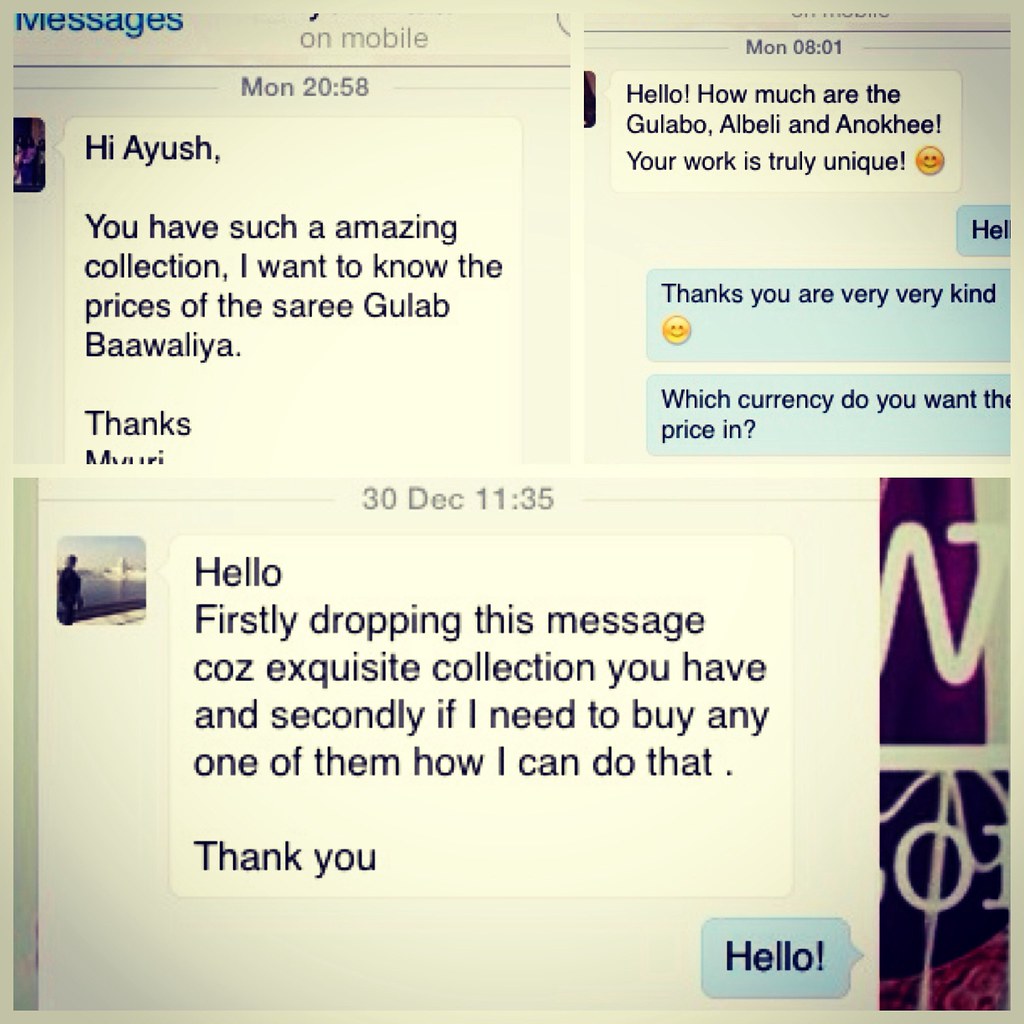The image is a screenshot of a social messaging app displaying multiple text exchanges about a unique collection of saris. There are three distinct conversation panels. The top-left panel is partially cut off but reads, "Messages on Mobile," and includes a message sent on Monday at 8:58 PM: "Hi Ayush, you have such an amazing collection. I want to know the price of the Sari Gulab Bawaliya. Thanks, Miri." The top-right panel contains another message asking, "Hello, how much are the Gulabo, Albeli, and Anoki? Your work is truly unique. 😊" The response in this panel says, "Hello. Thanks. You are very, very kind. Which currency do you want the price in?" The bottom panel, dated December 30th at 11:35, reads, "Firstly, dropping this message because of the exquisite collection you have. And secondly, if I need to buy any one of them, how can I do that? Thank you," followed by a response that simply says, "Hello." 

The screenshot showcases messages from admirers who are inquiring about the prices and purchasing details of various saris from Ayush’s collection, highlighting the admiration for the unique and exquisite nature of the designs.